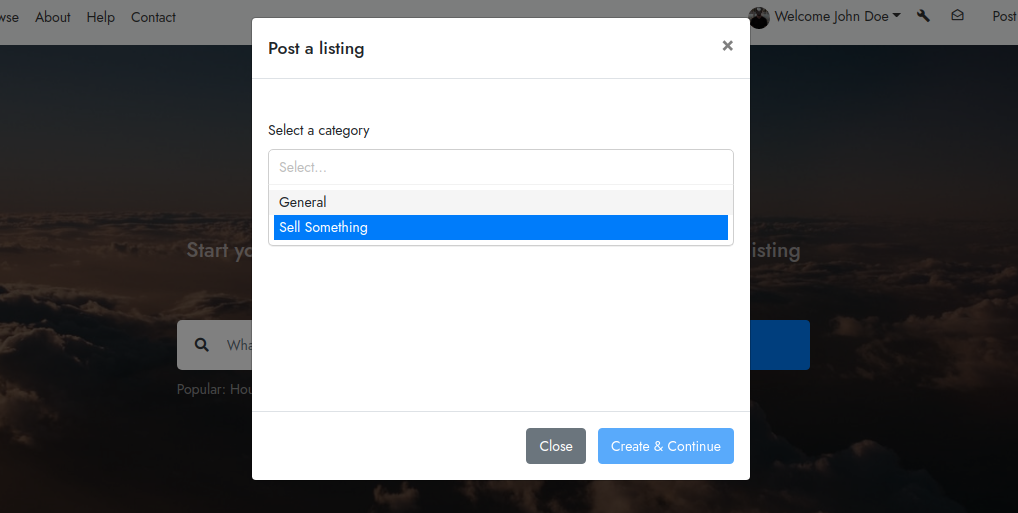In this image, we see a prominent pop-up box centered in the middle. At the top left of this pop-up box, there's bolded black text that reads "Post a Listing". To the far right at the top of the box, there's a gray-colored 'X' symbol. A thin black line beneath these elements separates the different sections of the pop-up.

In the middle section of the pop-up box, on the left side, it says "Select a Category". Below this prompt, there appears to be a dropdown chat box for category selection, currently displaying the word "General". Below this, a button highlighted with a blue background contains the phrase "Sell Something" in white text.

At the bottom right of the pop-up, there are two interactive buttons. The left button, with a black background, is labeled "Close". The right button, with a light blue background, is labeled "Create and Continue".

The background of the image reveals a webpage interface. At the top right corner of the webpage, the word "Post" is visible, accompanied by a mail icon and a wrench icon. Right next to these, there is a greeting "Welcome John Doe", alongside a circular profile picture to the left and a downward arrow to the right. At the top left of the webpage, the words "About," "Help," and "Contact" are also visible, indicating navigation options.